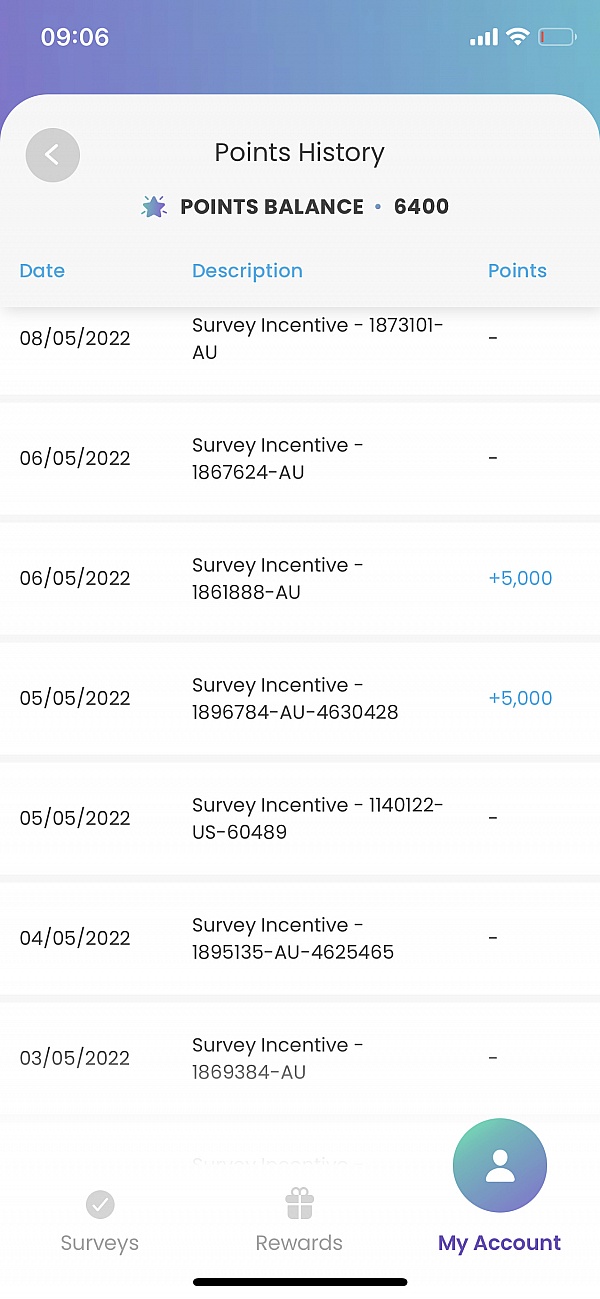This detailed caption enhances the clarity and structure of the original spoken description, providing a precise and comprehensive depiction of the image:

---

The image is a screenshot of a mobile phone screen displaying a points history summary for a survey rewards account. At the top, there's a status bar with a gradient from darker blue on the left to lighter blue on the right. The time displayed is 09:06. On the right side of the status bar, full signal for both cellular and Wi-Fi is indicated, but the battery icon shows low charge, marked by a thin red line on the left side of the nearly empty battery symbol.

Below the status bar, there's a section titled "Points History," highlighted with a small blue star icon next to it. The points balance displayed is 6400. The points history is organized in rows under three columns: Date, Description, and Points.

The entries include:

1. **08-05-2022** – "Survey Incentive-1873101-AU" – No points awarded (indicated by a dash).
2. **06-05-2022** – "Survey Incentive-1867624-AU" – No points awarded (dash).
3. **06-05-2022** – "Survey Incentive-1861888-AU" – Awarded **+5000** points (in blue).
4. **05-05-2022** – "Survey Incentive-1896784-AU-4630428" – Awarded **+5000** points (in blue).
5. **05-05-2022** – "Survey Incentive-1140122-US-60489" – No points awarded (dash).
6. **04-05-2022** – "Survey Incentive-1895135-AU-4625465" – No points awarded (dash).
7. **03-05-2022** – "Survey Incentive-1869384-AU" – No points awarded (dash).

Below the points history table, there are three navigation options in light gray:

1. **Surveys** – With a white checkmark inside a light gray circle.
2. **Rewards** – Depicted by a present icon in light gray.
3. **My Account** – Represented by a blue circle containing a white person icon. This section is highlighted with a black horizontal line below it.

The entire screen seems to be dedicated to tracking and displaying the points history and balance for someone actively participating in survey rewards.

---

This refined caption offers a vivid, step-by-step overview of the mobile screen's content, ensuring that all significant details are presented clearly.